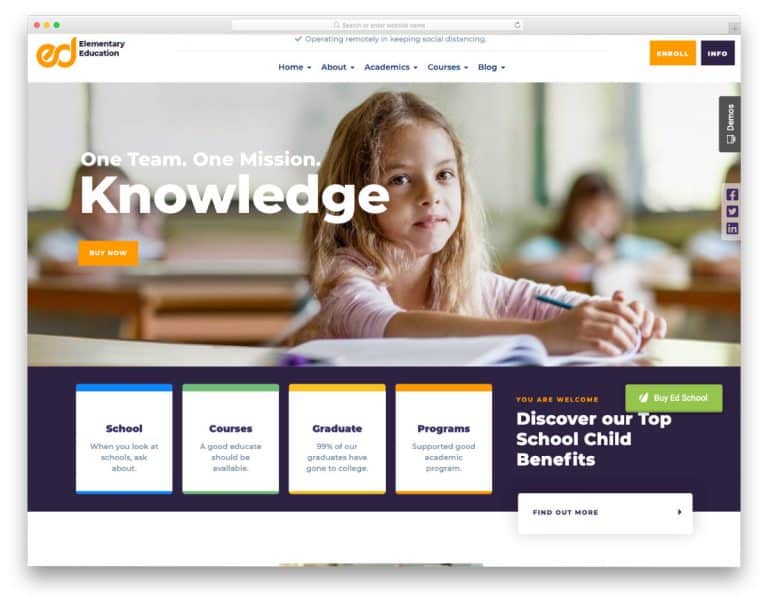A grainy screenshot of a website displayed on what appears to be a computer running macOS. At the top, there is a typical Mac navigation bar, hinting that it's a browser displaying a webpage. The page overall is not very clear, but several details are discernible. 

In the top left corner, there is an orange-ish logo accompanied by purple text reading "Elementary Education." Next to it, some additional text is present but unreadable due to the image quality. On the right-hand side of the logo are two buttons: an orange one with “Enroll” in white text and a purple one with “Info” in white text.

The website’s navigation menu spans the top of the page, listing tabs such as "Home," "About," "Academics," "Courses," and "Blog." 

Dominating the center of the screenshot is a banner image that features a young child sitting at a desk, holding a pencil and looking toward the camera. The banner has a motivational tagline in white text that says, "One Team, One Mission, Knowledge." Below this slogan is a yellow button with white text that reads "Buy Now."

Beneath the banner, there is a purple section displaying four different informational cards, but the text on these cards is grainy and hard to fully comprehend. The first card has a blue banner and appears to say "School. When you look at school ask about." The second card has a green banner and reads, "Courses. A good education should be available." The third card is yellow and mentions, "Graduate. 99% of our graduates have gone to college." The fourth card is orange and states, "Programs supported. Good academic program."

Underneath these, there is a statement in white text that says, "Discover Our Top School Child Benefits," accompanied by a green button that reads "Buy at School" and another white button with purple text that says "Find Out More."